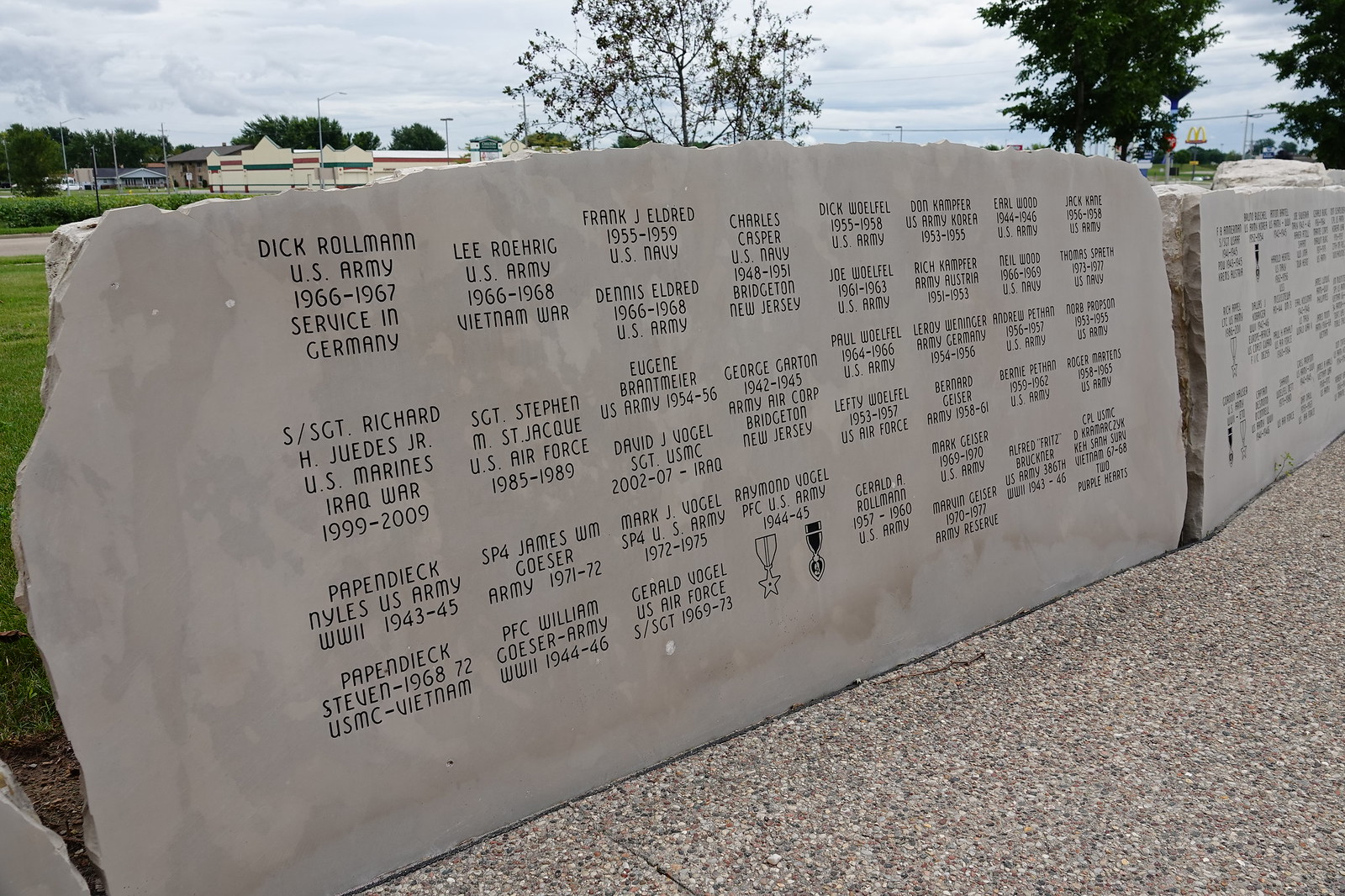The image depicts an outdoor scene with a cloudy, overcast sky. In the foreground, there is a slate gray monument consisting of two large stone tablets, each around four feet high, positioned along a sidewalk area. The monument honors servicemen, displaying the names, military branches, years of service, and locations of service for numerous individuals. One prominent name inscribed is Dick Rollman, U.S. Army, who served from 1966 to 1967 in Germany. The names are arranged in a grid layout, with an estimated 25 to 40 names visible. The background features a green lawn, several trees, a large building, and what appears to be a body of water in the distance. On the right side of the image, a McDonald’s arch is also visible.